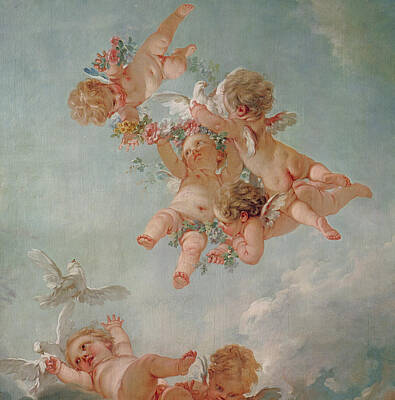The image is a detailed Renaissance-style painting of six cherubic baby angels floating in a bluish-gray sky filled with clouds. In the center, four cherubs with blondish-brown hair are depicted interacting closely; two are reaching upwards towards another cherub who appears to be descending, while one floats horizontally beneath them. Surrounding these central figures are white birds, including doves, and additional cherubs: one at the bottom center with only its head visible, and another to the left, floating on its back. All the cherubs have a pudgy, angelic appearance, some carrying flowers as they reach out towards each other and the birds. The serene atmosphere evokes a celestial scene filled with motion and harmony.